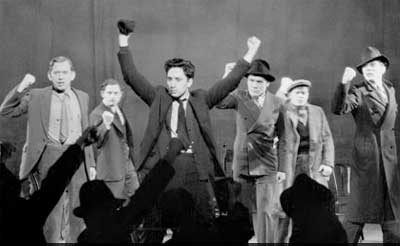In this black and white image, we witness a dynamic and striking scene featuring six men on a stage, all exuding a sense of triumph. The central figure, adorned in a suit and tie, commands attention with his dual fists raised high, holding an object in his right hand. Flanking him, two men to the left and three to the right, all equally attired in suits and ties, mirror his stance with one raised fist each. Three of these men also sport hats, adding a distinguished touch to their appearance. Below the stage, a silhouetted crowd observes, many mirroring the raised fists of the men on stage, amplifying the atmosphere of unity and victory within the scene.